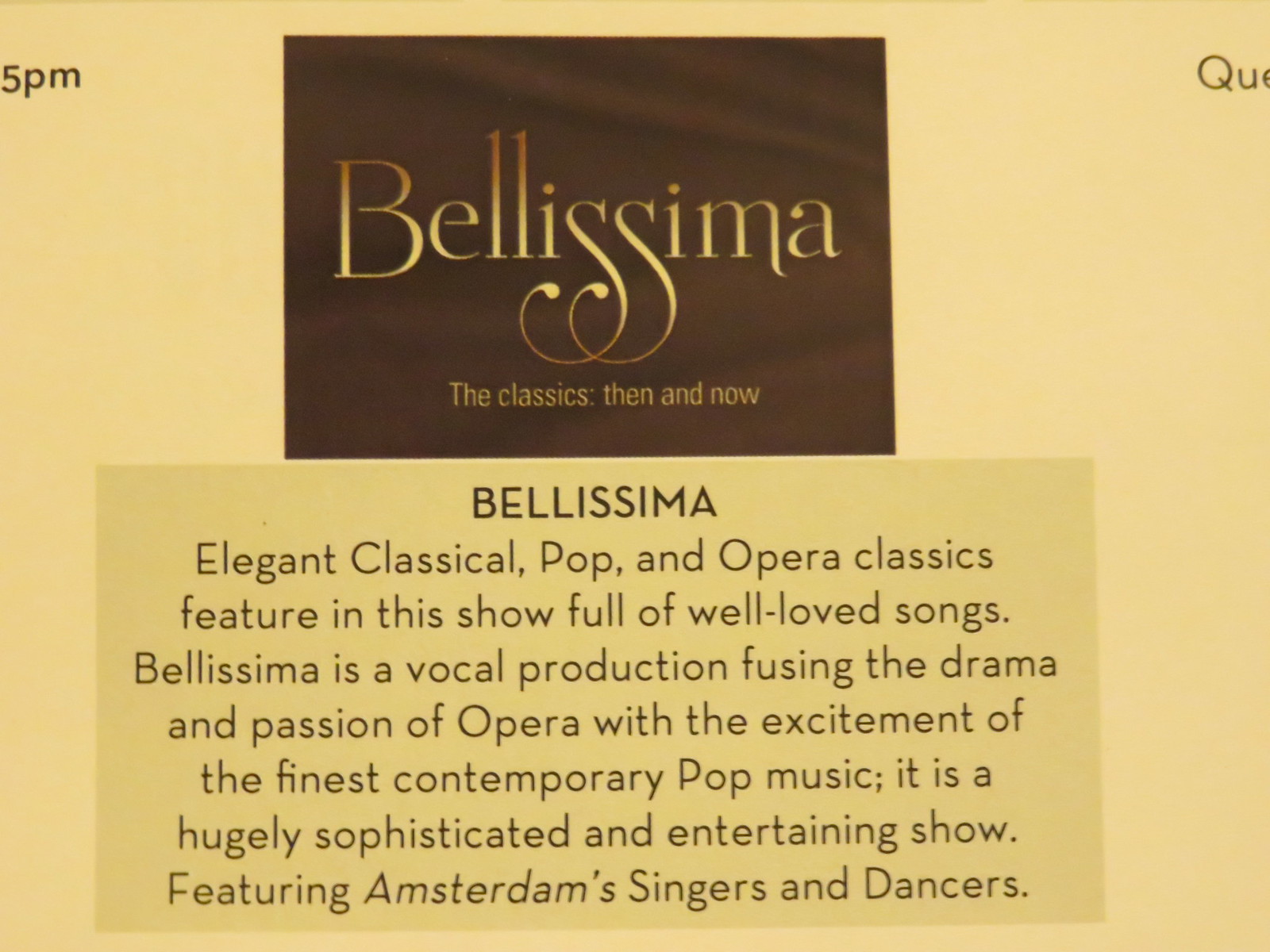This image is an elegantly designed advertisement for an event named "Bellissima," written in a very ornate golden font against a brown background with a yellowish-tan overlay. Positioned at the top left, the event's time is 5 p.m. The subtitle "The Classics, Then and Now" follows directly underneath in the same golden font. Below this title, a detailed description highlights that the show is an elegant blend of classical pop and opera classics, featuring well-loved songs. The description emphasizes that "Bellissima" is a vocal production that fuses the drama and passion of opera with the excitement of the finest contemporary pop music. Additionally, it's noted that the show is not only sophisticated and entertaining but also features singers and dancers from Amsterdam. Prominently showcased at the top of the image, the "Bellissima" logo has a fluid, embellished design, with exaggerated S's that swoop down elegantly. The entire layout suggests a sophisticated marketing piece, possibly an excerpt from a program or magazine distributed at an operatic event.